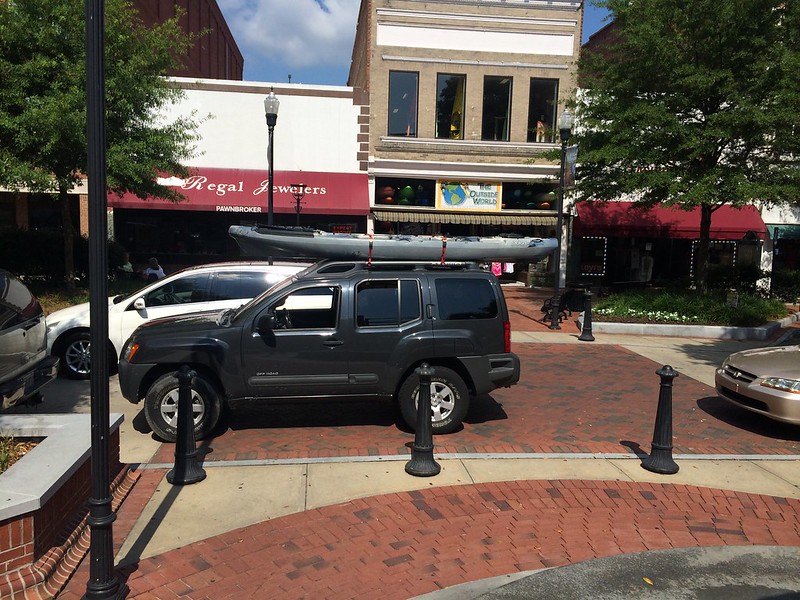The image captures a charming, decorative street scene featuring brick roads and sidewalks. In the foreground, a sidewalk with a brick pattern runs parallel to the street. Multiple parked cars line the road, including a distinctive gold car and a black SUV with a kayak secured on top by two red clips. On the opposite side of the street, a picturesque row of shops enhances the lively atmosphere. To the left stands Regal Jewelers, marked by its white and red façade. The central store, taller than its neighbors and adorned in a stone color with numerous windows, appears to have a sign that possibly reads "The Outside World." The store to the right mirrors Regal Jewelers' red and white design. Lush plants and trees interspersed along the brick sidewalk contribute to the area's scenic beauty.